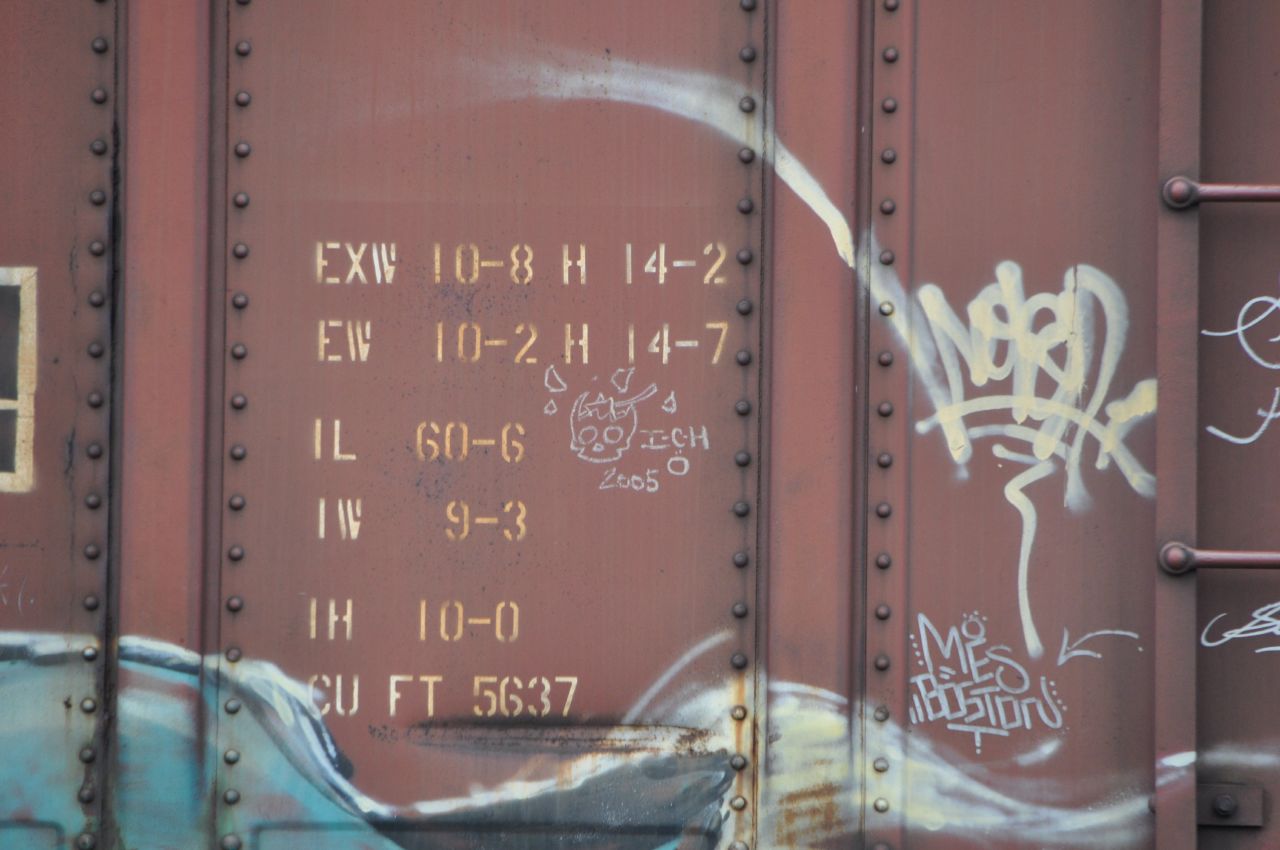The photograph captures the side of a rusted, light red metal structure, likely a freight train car or shipping container, filling the entire landscape-oriented frame. Prominently, the exterior includes bolts or rivets arranged in columns, suggesting heavy-duty construction. A ladder is visible on the right side, hinting at access to the roof. Scattered across the surface are various numbers and letters, such as "EXW 10-8 H 14-2" and "cubic feet 5637," indicating capacity or identification marks. Notably, graffiti adorns the metal wall: white or cream-colored tags with some text possibly reading "MES Boston" and a partially obscured illustration featuring what appears to be a blue wave alongside a cracked skull marked "ICH 2005." This vivid display of urban artistry coexists with the utilitarian and weathered character of the structure.